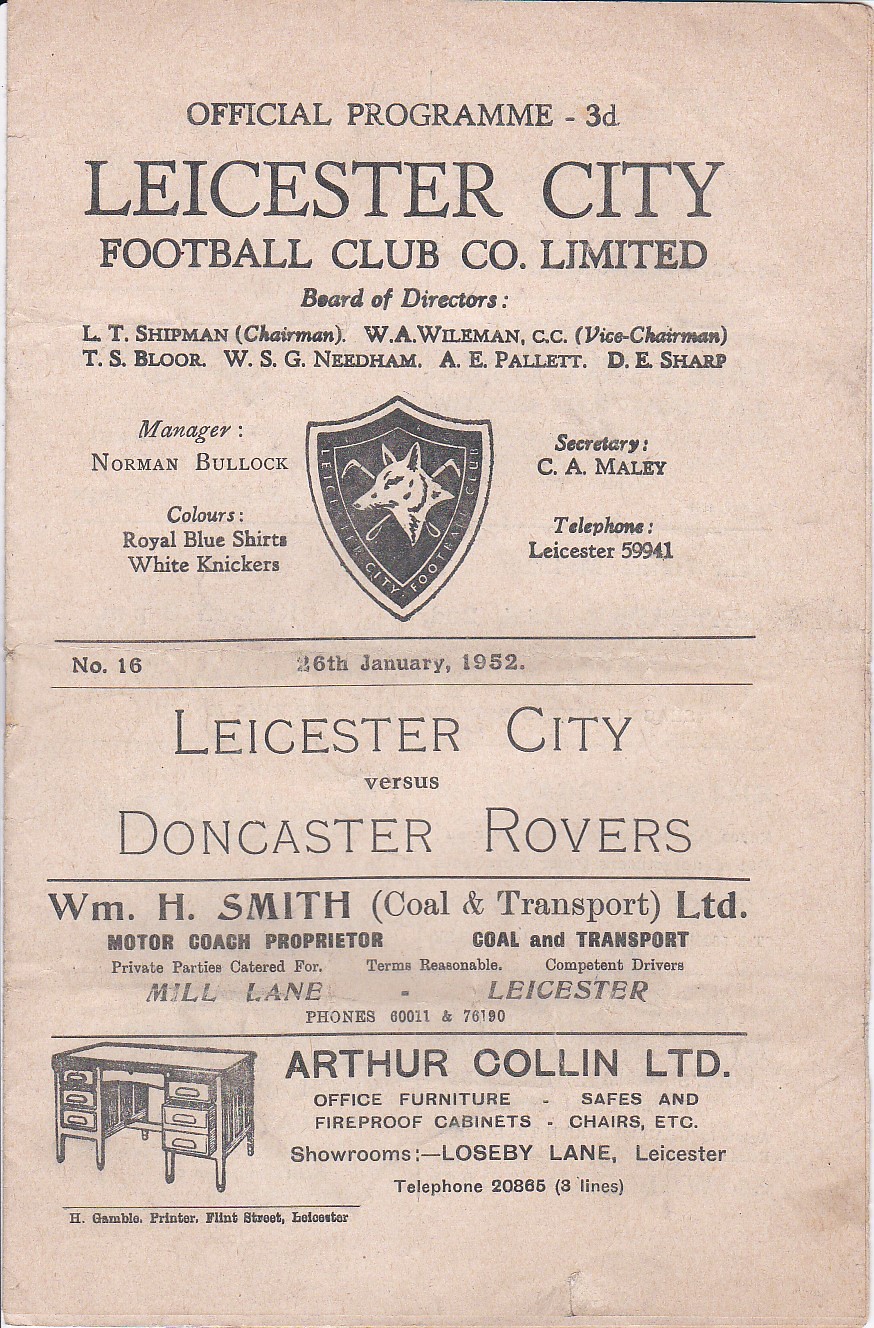The image is of an aged, official program for Leicester City Football Club Ltd., dated 26 January 1952. The background is a worn beige color, presumably having faded from white over time, with black text centered on the page. At the top, in prominent black print, it reads "Official Programme - 3D," followed by "LEICESTER CITY FOOTBALL CLUB LIMITED." Below, the Board of Directors is listed, including L.T. Shipman as Chairman and W.A. Wileman CC as Vice Chairman, among others. The logo of the Leicester City Football Club, resembling a dog or wolf with crisscrossed items behind it, possibly golf clubs, is situated centrally. Additional details include the managers' names, the secretary, and a telephone number (Leicester 59941). Advertisements for WH Smith Ltd. and Arthur Collin Ltd., the latter featuring a visual of a desk, appear at the bottom. The program is marked as number 16 and notes the match between Leicester City and Doncaster Rovers. The club colors are noted as royal blue skirts and white knickers.